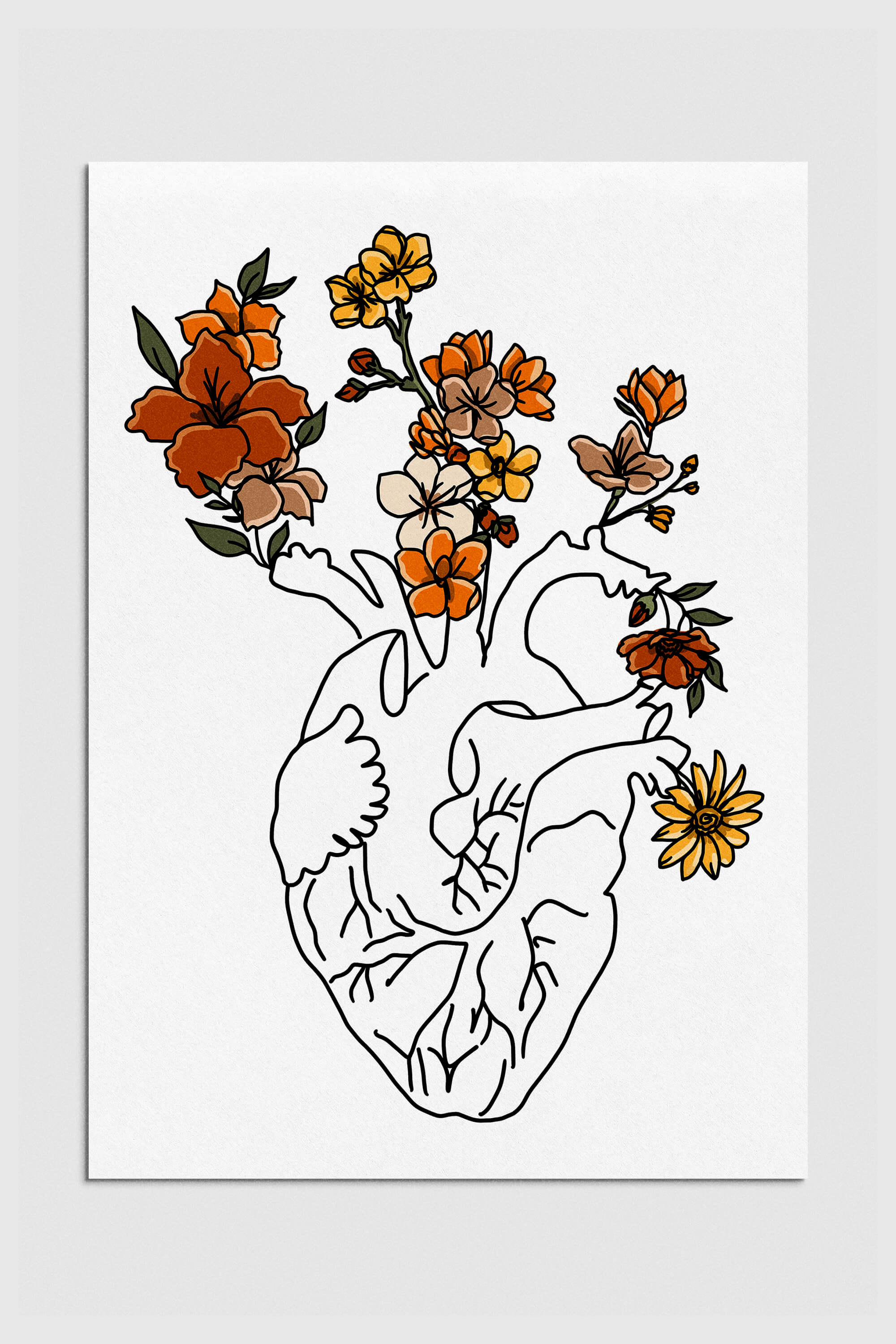This artwork is a black-and-white sketch of a human heart, detailed with vein and artery lines as well as small capillaries. Emerging from various parts of the heart's top and sides, colorful flowers sprout, enhancing the contrast. The flowers, resembling daisies, display a sophisticated palette of muted yet varied colors including dark red, brown, yellow, beige, orange, and light pink. Among the blooms, a few small green leaves and buds add to the intricate depiction. Presented on an unframed white canvas, the piece hangs against a beige wall, combining simplicity and dramatic flair with its juxtaposition of monochrome and subdued, yet vibrant, floral elements.